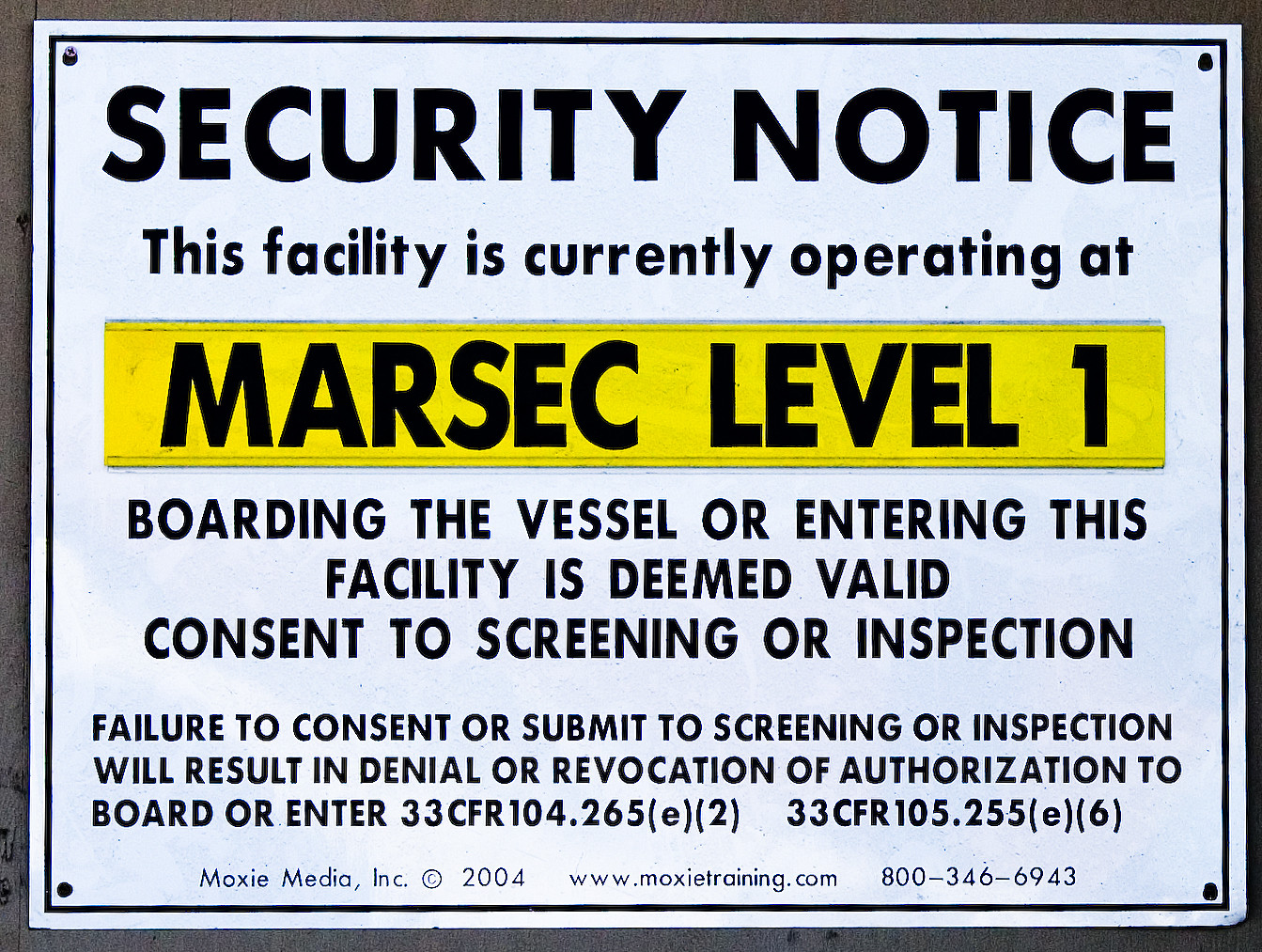The image features a rectangular metal sign mounted on a wall, with visible metal screws securing it at each corner. The sign has a white background encased by a thin black border. At the top center, in bold black font, it reads "SECURITY NOTICE." Below this, the sign states, “This facility is currently operating at,” followed by a yellow horizontal box with bold black text inside declaring “MARSEC Level 1.” Further down, the sign continues in black lettering, “Boarding the vessel or entering this facility is deemed valid consent to screening or inspection.” It then adds in smaller font, “Failure to consent or submit to screening or inspection will result in denial or revocation of authorization to board or enter.” The applicable laws are listed as “33 CFR 104.265(e)(2)” and “33 CFR 105.255 (e)(6).” At the bottom, there is a line of text with the copyright information: “Moxie Media, Inc., ©2004, www.moxietraining.com, 800-346-6943.”